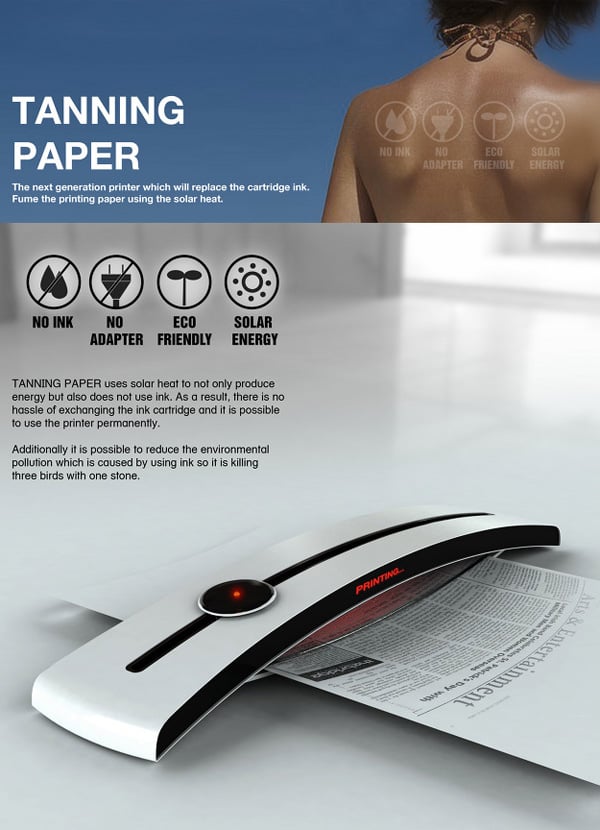The image is a detailed advertisement for an innovative product called "tanning paper." The ad features a sleek, narrow, and slightly curved printer that is primarily white with accents of black and red. Positioned at the top of the image, there's a blue border that spans across the page, and within it is a compelling visual of a woman with bushy brown hair viewed from behind, her bare back exposed, evoking a sense of natural simplicity.

Prominently displayed on the top left in the white text, "tanning paper" introduces the product. Below this, a series of emblems illustrate its unique selling points: no ink, no adapter, eco-friendly, and solar energy. These emblems are set on a white background with black icons and text. A detailed paragraph explains that the tanning paper uses solar heat to prime the paper, eliminating the need for ink cartridges and thereby reducing environmental pollution—a triple benefit of convenience, sustainability, and cost-efficiency.

Towards the lower portion of the image, the advertisement elaborates on how this next-generation printer leverages solar energy both for power and the printing process itself. The blue with white writing makes it clear that this printer offers a revolutionary approach to reducing environmental waste. The text blocks and images point to a user-friendly experience, supported by a manual and a remote control featured on the ad.

Overall, the intricate details and modern aesthetics of this advertisement highlight the cutting-edge technology and eco-conscious design of the tanning paper printer, emphasizing its role as both an innovative and environmentally friendly solution.